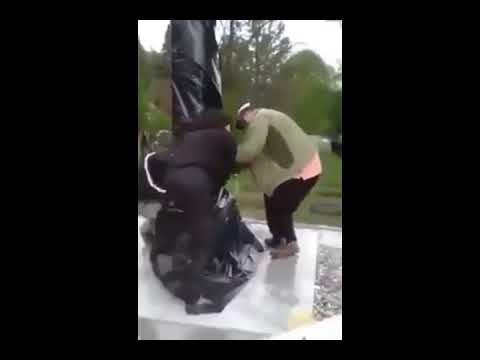In the image, a very large man, possibly wearing welding goggles on his head, stands on a grey stone-tiled platform outdoors in the rain. The platform's floor is wet, reflecting the dreary weather. The man is dressed in a grey coat and black pants. He seems to be working on something suspended from above, likely a black tarp-like material hanging from the top edge of the image. Surrounding him is a backdrop of lush green trees, with a sliver of grey sky visible. To the left, another man similarly dressed in dark colors appears to assist with the task. Despite the image's blurriness, both men are clearly engaged in their work on the platform amidst the outdoor setting.